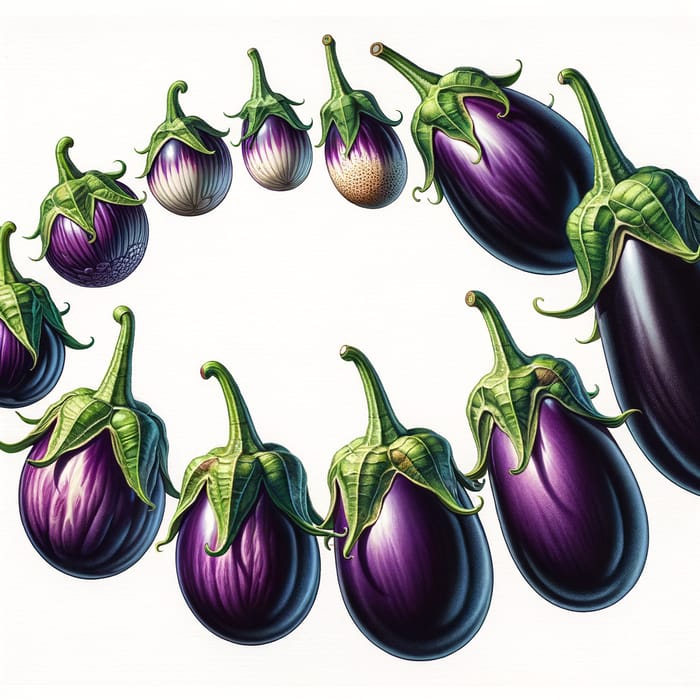This illustration showcases 11 to 12 eggplants arranged in a circle against a white backdrop. The eggplants, varying in size and patterns, are depicted in a gradation from smaller to larger as they form the circle. Some eggplants are small with a speckled white base and purple top, while others have a white-streaked base melding into purple. A few are solid purple and either smooth or ridged. Additionally, there are longer, darker purple eggplants among them. Each eggplant is crowned with a green stem and triangular leafy tops, resembling small green crowns. Despite the differing shapes and textures—some being rounder and others more elongated—all the eggplants have a smooth, shiny appearance, accentuated by a spotlight that casts subtle highlights and shadows. This careful arrangement of the eggplants displays a harmonious yet diverse collection, encircling the frame elegantly.